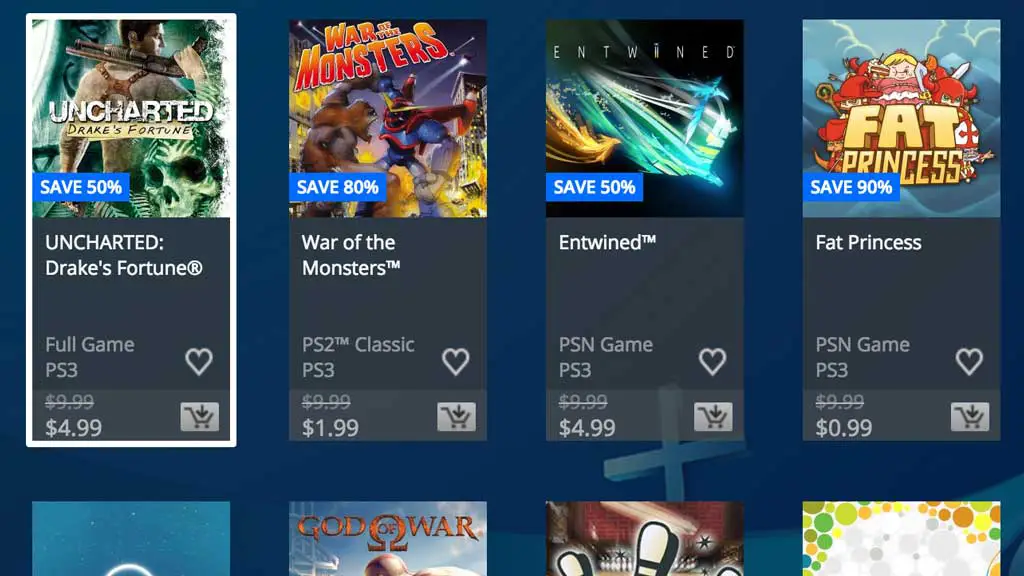The image depicts a low-resolution, somewhat pixelated webpage showcasing multiple game titles. The quality is quite poor, making the image blurry and fuzzy. On the top left corner of the webpage is the game titled "Uncharted: Drake's Fortune." The cover image displays the back view of a man, with a skull visible near the bottom right. Text below the cover indicates "Full Game PS3." The original price of $9.99 is crossed out, showing a discounted price of $4.99 beneath it.

To the right of this game is another title called "War of the Monsters." The cover features an ape on the left side and a robot on the right. Below this cover, the text reads "PS2, TM Classic, PS3," with the price listed as $9.99.